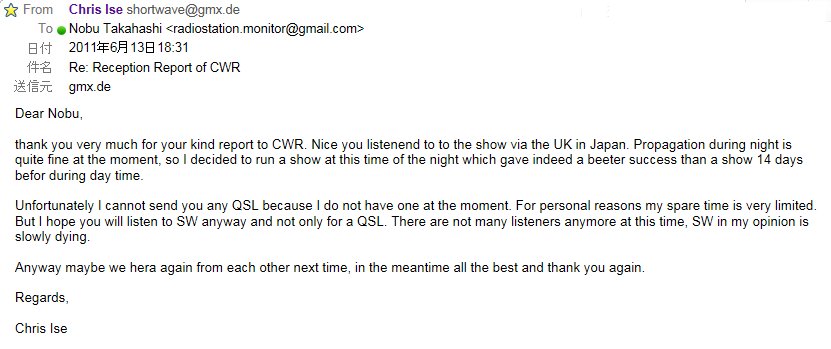The image depicts a white-background screenshot of an email from Chris Ice (shortwave@gmx.de) to Nobu Takahashi (radiostation.monitor@gmail.com). The email was sent on June 13, 2011, at 18:31. The subject line is "Regarding Reception Report of CWR." There are some Chinese or Japanese characters in the header, particularly around the date and email fields, which indicate additional options like BCC. The body of the email starts with "Dear Nobu," and thanks Nobu for his reception report to CWR. Chris appreciates Nobu's effort in listening to the show via the UK and Japan. Chris explains that nighttime propagation is currently favorable, which led to the decision to broadcast at night, resulting in better success compared to a daytime show held 14 days earlier. He apologizes for not being able to send a QSL card due to personal time constraints but encourages Nobu to continue listening to SW. He also mentions the declining number of SW listeners and expresses hope to hear from Nobu again. The email concludes with "Regards, Chris Ice." There is a yellow star icon at the top left indicating a marked or important message, and the presence of these intricate details emphasizes the careful consideration given to Nobu's reception report.